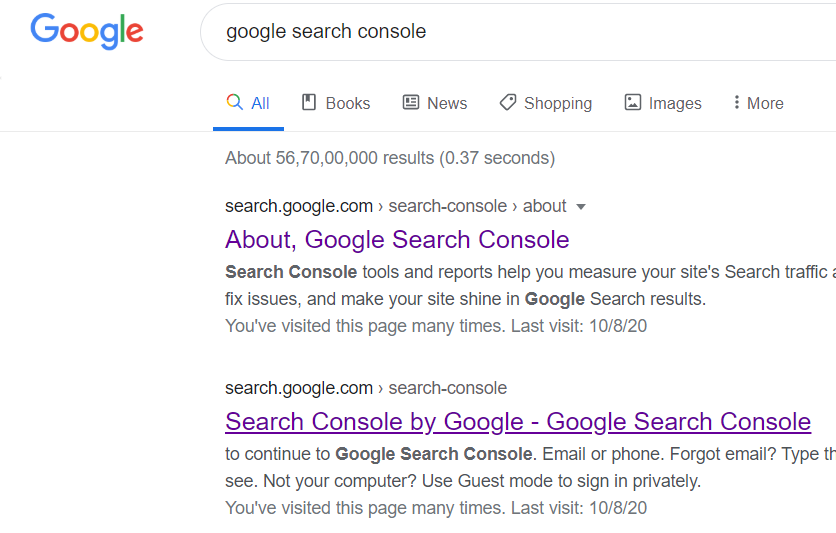The image depicts a Google search results page. The interface shows the recognizable Google logo at the top, followed by the search query "Google Search Console" in the search box. Below the search box, the navigation options are displayed, with "All" highlighted in blue, and other options such as Books, News, Shopping, and Images listed in sequence on a white background.

The first search result is a link to the Google Search Console's main information page. The title is displayed in prominent purple lettering, reading "About Google Search Console," and is followed by a description in black text: "Search Console, Tools and Reports help you measure your site's search traffic, fix issues, and make your site shine in Google search results." A note indicates that the user has visited this page multiple times, with the most recent visit on October 8th, 2020.

The second search result also relates to Google Search Console, titled "Search Console by Google - Google Search Console," shown in the same purple and underlined for emphasis. The snippet beneath it provides login instructions for continuing to Google Search Console, with options to enter an email or phone number, and a reminder about guest mode for private sign-in. Similar to the first result, it notes that the user has visited this page frequently, with the last visit also being on October 8th, 2020.